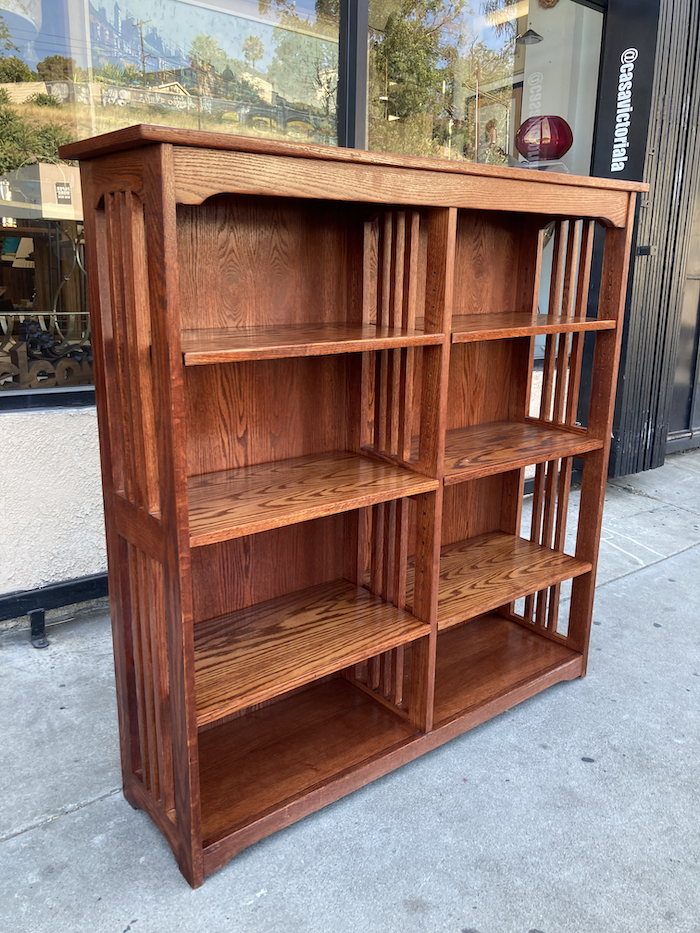This photograph captures a large, freestanding shelving unit made of oak, stained a darker shade that showcases the wood grain. The unit is divided into two sections, each containing four shelves, with a total of eight shelves—not including an additional top surface that can be used for displaying items such as planters. The shelving unit is situated on a sidewalk in front of a store with windows, though the inside details are obscured by reflections and furniture. The visible storefront bears the sign "Casa Victoria." The unit's structure includes a central divider which segments the shelves, preventing items from spanning the full width of the unit. Despite resembling a dresser at a glance, the piece serves as a detailed, multi-shelved bookcase or cabinet, standing prominently against the backdrop of the storefront.